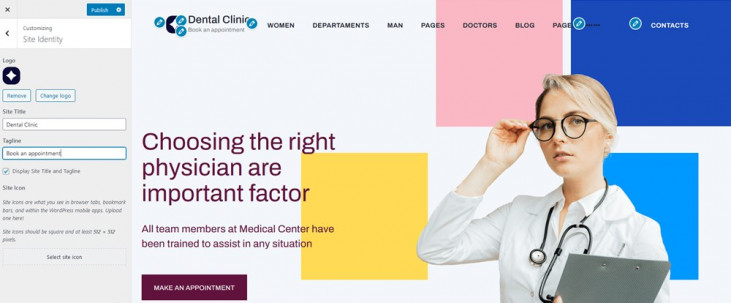This rectangular image appears to be a screenshot. On the left side, there is a gray box with blurred text. Within this gray box, a white banner prominently displays the words "Customizing Site Identity." Below the banner, there are two white boxes outlined in blue, labeled "Remove" and "Change Logo." The "Site Title" is identified as "Dental Clinic."

To the right of the gray box, the background turns white. In the upper-left corner, the text "Dental Clinic" is visible. Further to the right, there is a horizontal navigation bar with menu options: "Women," "Departments," "Man," "Pages," "Doctors," "Blog," and "Page." In the upper-right corner, the word "Contacts" is listed.

Beneath the navigation bar, a prominent line of dark burgundy text reads: "Choosing the right physician are [sic] an important factor. All team members at the medical center have been trained to assist in any situation." Below this text, there is a box with an option to "Make an Appointment."

On the right side of the image, there is a photo of a blonde woman. She is wearing a stethoscope, holding a clipboard, and has dark-rimmed glasses.